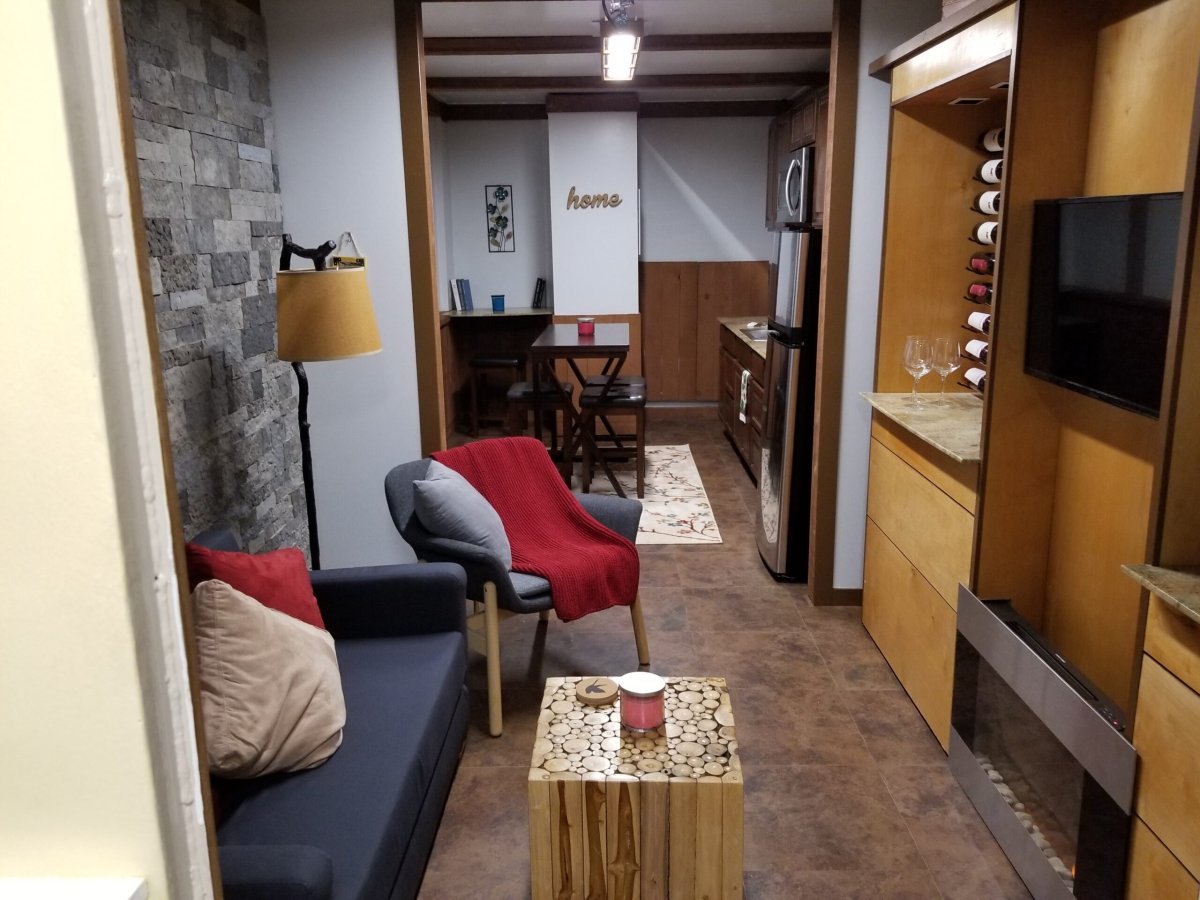This lifestyle image captures a meticulously staged, narrow living space that could be part of an apartment or home, possibly intended for Airbnb rental or sale. The room features a modern blue couch adorned with tan and red pillows positioned on the left, coupled with a lamp that has a yellowy cream lampshade, possibly crafted from a stick. Adjacent to the couch is a matching modern blue chair draped with a red throw. A boxy bamboo table sits at the center atop tiled flooring. Along the right wall, a built-in wooden unit houses a flat-screen TV above a small fireplace, flanked by wine bottles and clear wine glasses. In the same area, there's a gray chair with a gray pillow and another red blanket. The foreground extends into a kitchen, showcasing a silver refrigerator, wooden countertops, and a bench-style dining table accompanied by wooden chairs. A white Persian rug adds a touch of elegance to the space. On the wall in the background, a sign reads "Home," and overhead, fluorescent lighting illuminates the room. Despite the modern decor, the TV appears slightly small and close to the couch, suggesting a cozier, perhaps older setup.